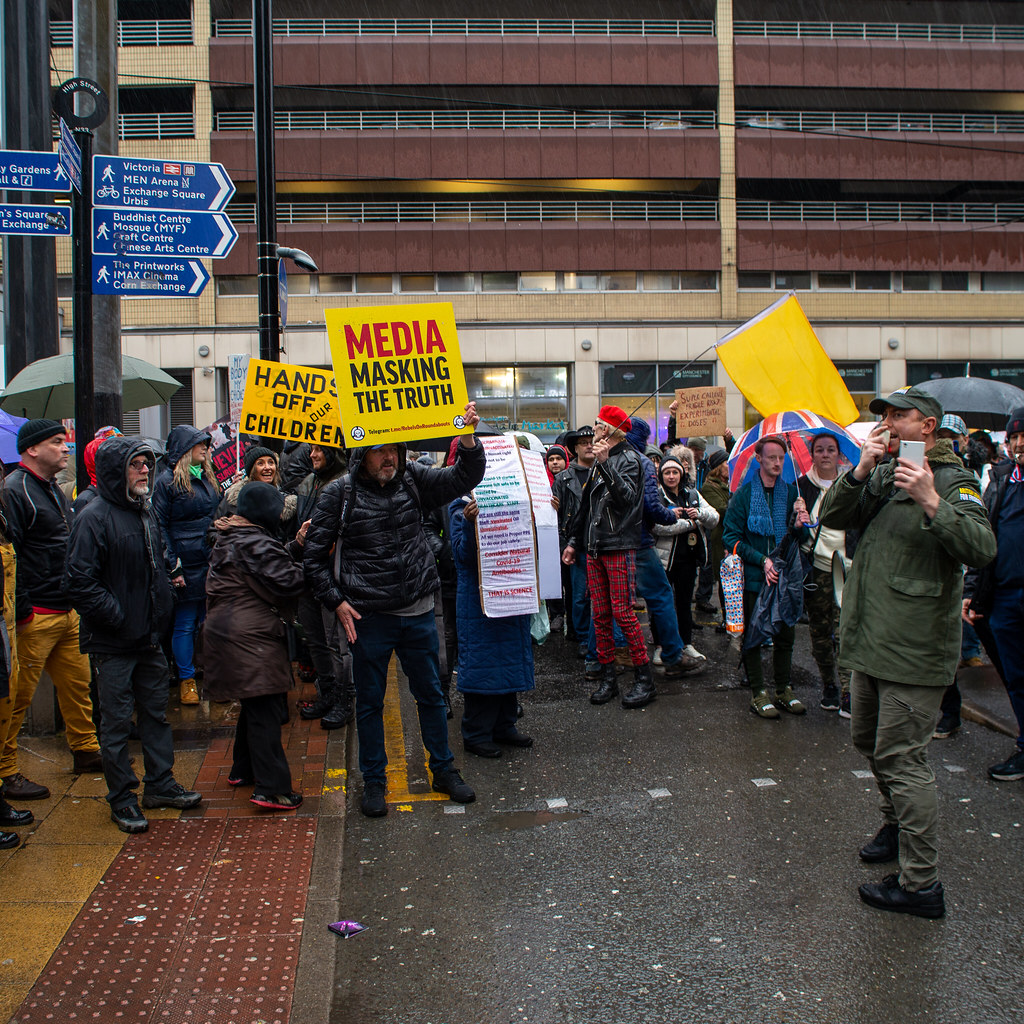In this image, a large group of protesters gather at a city intersection on a rainy, overcast day. The wet ground and the array of jackets, hoods, and umbrellas testify to the recent rainfall. Signs in the background include "Victoria Men Arena," "Exchange Square," "Buddhist Center," and "Mosque." Prominently, people in the crowd hold signs with messages like "Hands Off Our Children" and "Media Masking The Truth." One man, standing near the camera in a green jacket, holds a phone and a voice amplifier, seeming to address the crowd. A noteworthy pair under a British flag umbrella adds to the palette of umbrellas seen throughout the scene. The background features a large building, possibly a parking garage, adding an urban backdrop to the protest. The crowd, consisting of both men and women, stands on the street and sidewalk, some carrying signs not fully readable in the photo.